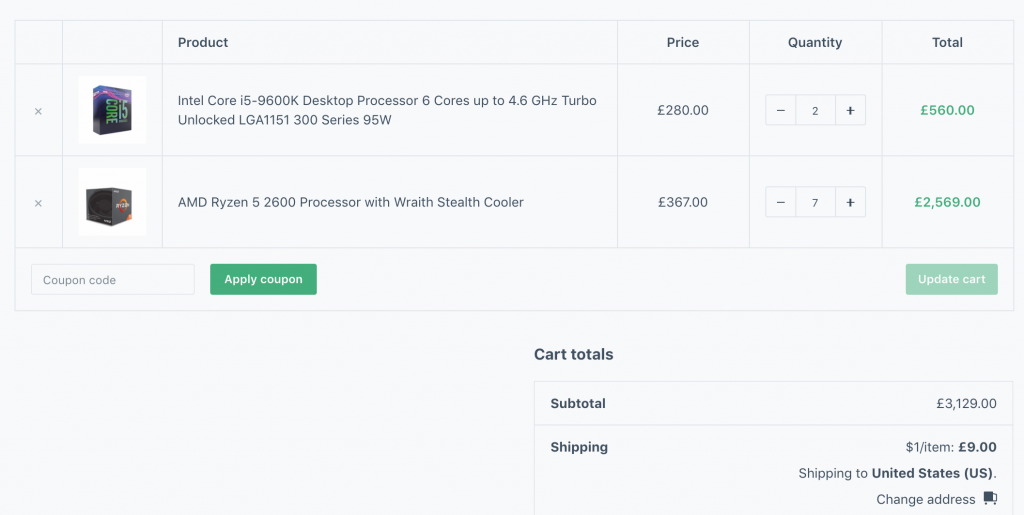**Shopping Cart Screenshot**

The image is a detailed screenshot of an online shopping cart interface. At the top, there is a table with six columns: Product, Image, Price, Quantity, Total, and a category unspecified in the voice note. The cart contains two rows of items:

1. **Item 1**: The first product depicted with a small image of its box is an "Intel Core i5-9600K Desktop Processor". This processor features six cores and can achieve speeds of up to 4.6 GHz with Turbo Boost. It is compatible with LGA1151 300 series motherboards and has a thermal design power (TDP) of 95 watts. The price is listed as £280, and the quantity selected is two, bringing the line total to £560.
   
2. **Item 2**: Directly below, the second product shown is an "AMD Ryzen 5 2600 Processor" which comes with a Wraith Stealth cooler. The price for this item is £367, and a quantity of seven is selected, totaling £2569.

Below these items, there is a section where the user can input a coupon code to apply discounts to their order, accompanied by an "Update Cart" button. 

Towards the bottom of the screenshot, the cart subtotal is displayed as £3129. The shipping cost is specified at £1 per item, amounting to £9 for this order. Shipping is indicated to be directed to the United States (US), with an option available to change the delivery address.

A "Proceed to Checkout" button is presumably present but not mentioned in the voice description.